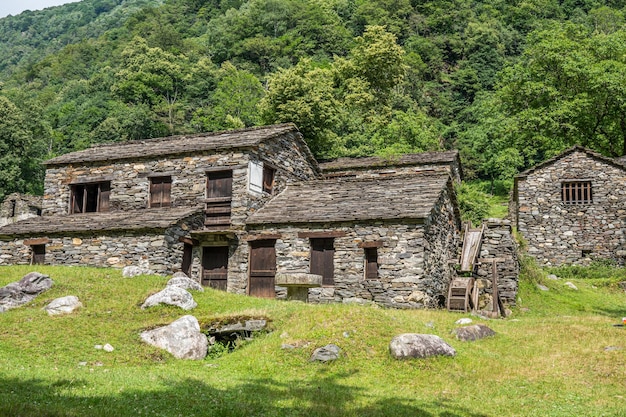This photograph captures a scene of two ancient stone buildings set in a rugged, hilly landscape typical of the Irish countryside. Nestled into the side of a steep, forested hill that rises beyond the frame, the primary structure is a partially two-story stone cottage. Its roof shows severe disrepair, and many of its windows are either missing or boarded up, with wooden shutters and doors accentuating the weathered look. To the right of this main building, there's a secondary stone structure, likely a barn, featuring barred windows and partly boarded-up openings that appear to use fence posts. Between the buildings, a small, dry water wheel is visible, partially embedded in the ground. The rocky front yard is strewn with large boulders and patches of grass, enhancing the rugged charm of the scene.